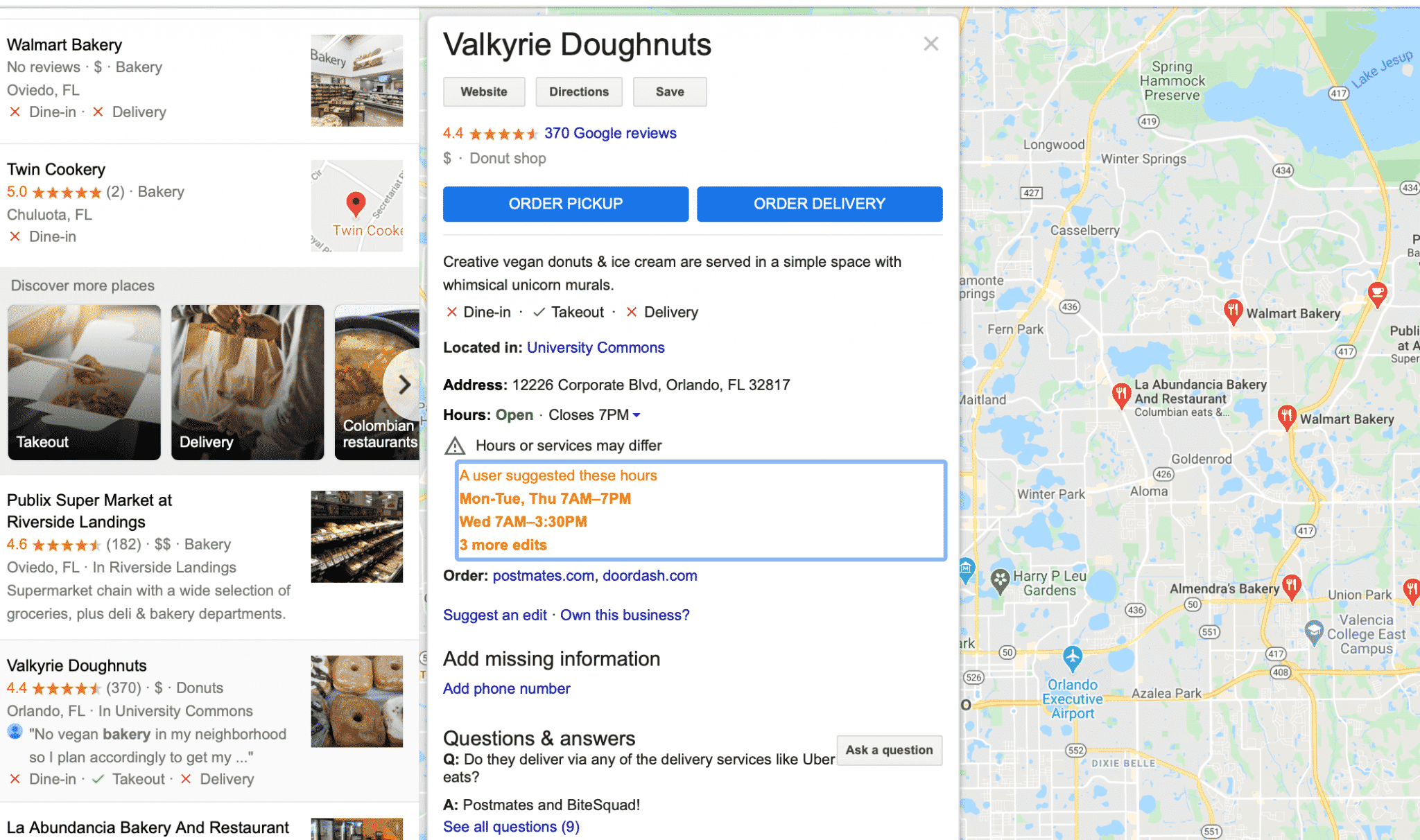This detailed caption describes a composite image made up of three smaller, vertical rectangle images arranged horizontally to form a single longer rectangle. 

The first image on the left features several snapshots of various place names and their logos, including "Walmart Bakery," "Twin Cookery," "Takeout Delivery," "Colombian," "Public Supermarket," "Riverside Landings," and "Valkyrie Donuts." Although the names are clearly visible, one name at the bottom is partially cut off.

The central image highlights "Valkyrie Donuts," which appears to be the selected option. At the top, navigation options such as "Website," "Directions," and "Save" are displayed, along with actionable buttons "Order Pickup" and "Order Delivery" in blue with white text. The description reads, "Creative Vegan Donuts and Ice Cream are served in a simple space with whimsical unicorn murals," and notes that the service options are limited to takeout, without dine-in or delivery. It also mentions the location as "University Commons," providing further details about the establishment.

The final image on the right features a map showcasing the various locations mentioned, with corresponding markers that align with the place names listed in the leftmost image.

Together, the three images provide a comprehensive visual and informational overview of Valkyrie Donuts, combining business names, detailed descriptions, service options, and geographical information.